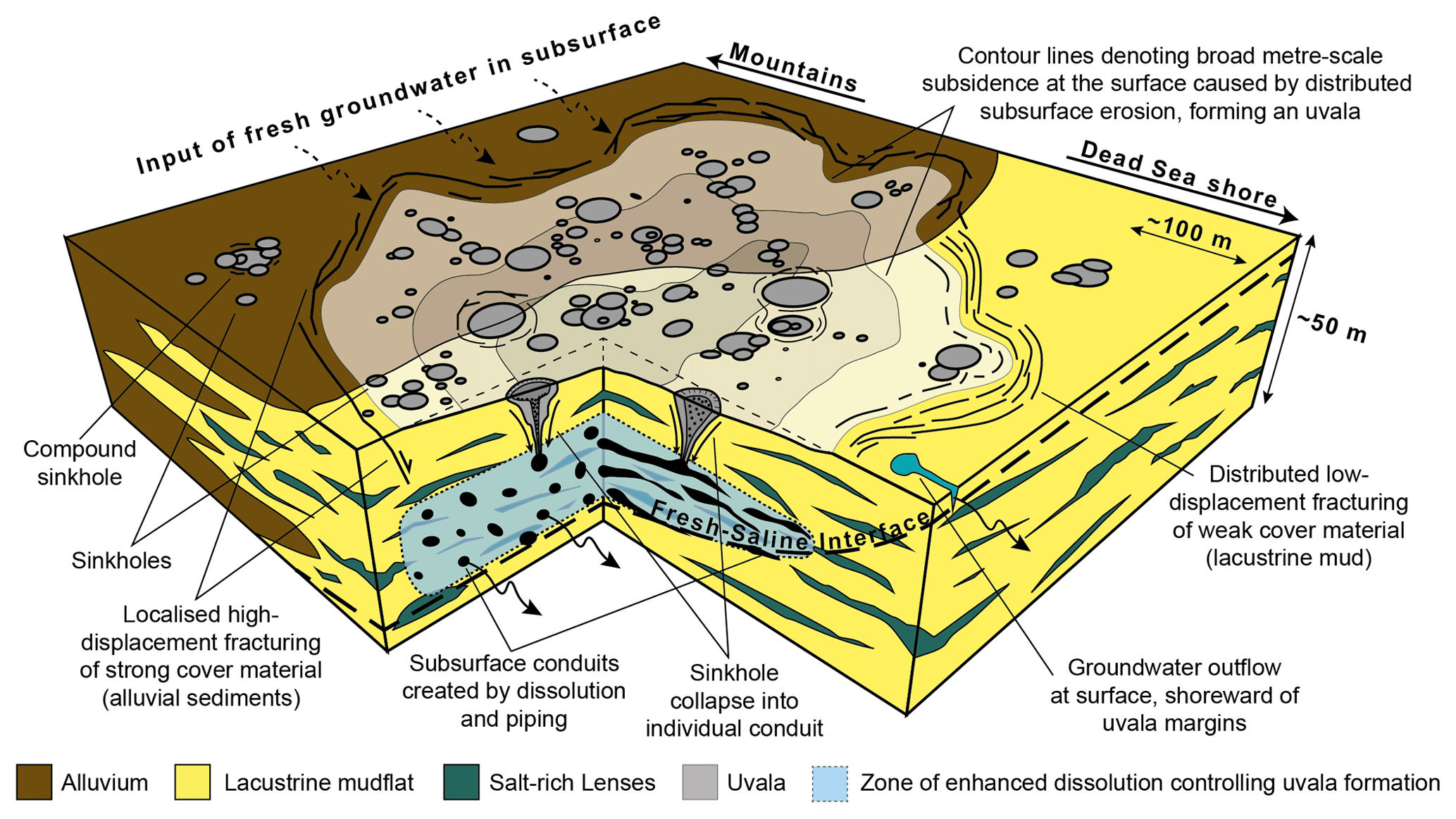This image is a detailed, landscape-mode diagram, resembling a complex textbook illustration, depicting a cross-section of the Earth's crust from mountains to the Dead Sea shore. With a predominant brown shade indicating alluvium, transitioning to light brown, yellow lacustrine mud flats, and intermittent areas of blue representing groundwater, the diagram is rich in labels and explanations. It features contour lines showing broad metro-scale and meter-scale subsidence caused by distributed subsurface erosion, forming an uvula.

The top left of the diagram highlights the "Input of fresh groundwater in subsurface," with arrows pointing towards the mountains and the Dead Sea shore. The central part of the diagram shows the subsurface, detailing complex geological formations such as compound sinkholes and subsurface conduits created by dissolution and piping, some labeled as showing a cross-section of 50 and 100 meters. Key features such as "fresh saline interface," "compound sinkhole," and "localized high displacement fracturing of strong cover material (alluvial sediments)" are clearly marked.

Additionally, the diagram employs a color-coded index to describe various sediment types and geological features: brown for alluvium, yellow for lacustrine mud flats, green for salt-rich lenses, silver for uvula, and light blue for the zone of enhanced dissolution controlling uvula formation. The bottom of the diagram contains groundwater outflow and points to a distributed low displacement fracturing of weak cover material identified as lacustrine mud. Each feature is meticulously labeled to elucidate the subterranean processes shaping the landscape.